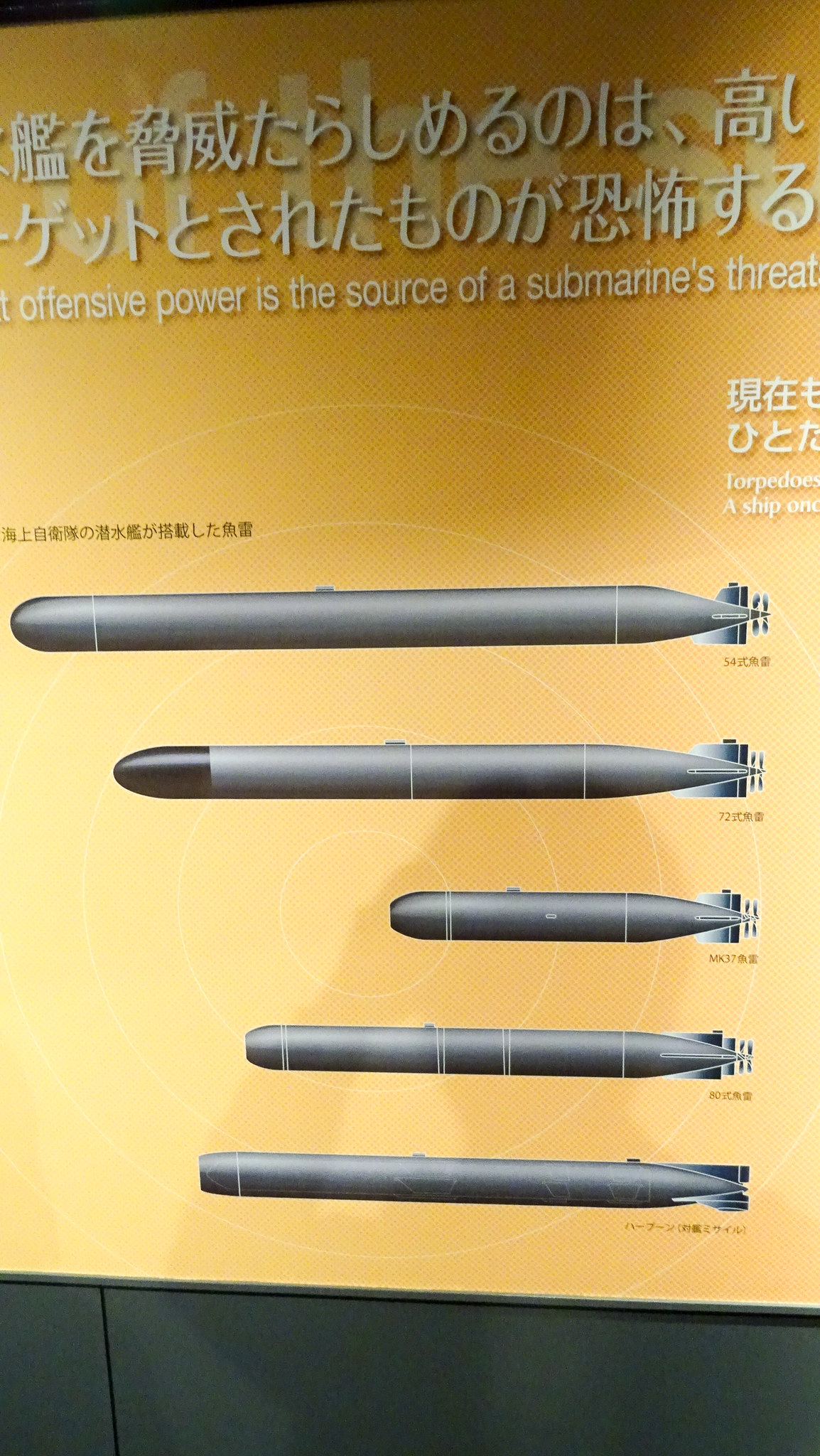The image depicts a digitally created poster showcasing five distinct Japanese torpedoes arranged vertically, each varying in length. The torpedoes are positioned with their propellers on the right side and their heads facing left, suggestive of an underwater movement. The backdrop is a halftone gradient background in varying shades of yellow, darker at the top and lighter at the bottom, with sonar-like radar rings emanating from the bottom center. The poster has an orange hue and features white text in Japanese at the top, accompanied by an English translation that reads, "Offensive power is the source of a submarine's threat." Additional text on the right side of the poster includes the word "Torpedoes," although it appears partially cropped. The torpedoes themselves are silver with guiding fins, and each has a distinct shape, with one notably featuring a flat head. This detailed display likely serves a marketing or informational purpose, emphasizing the diversity and design of Japanese submarine weaponry.